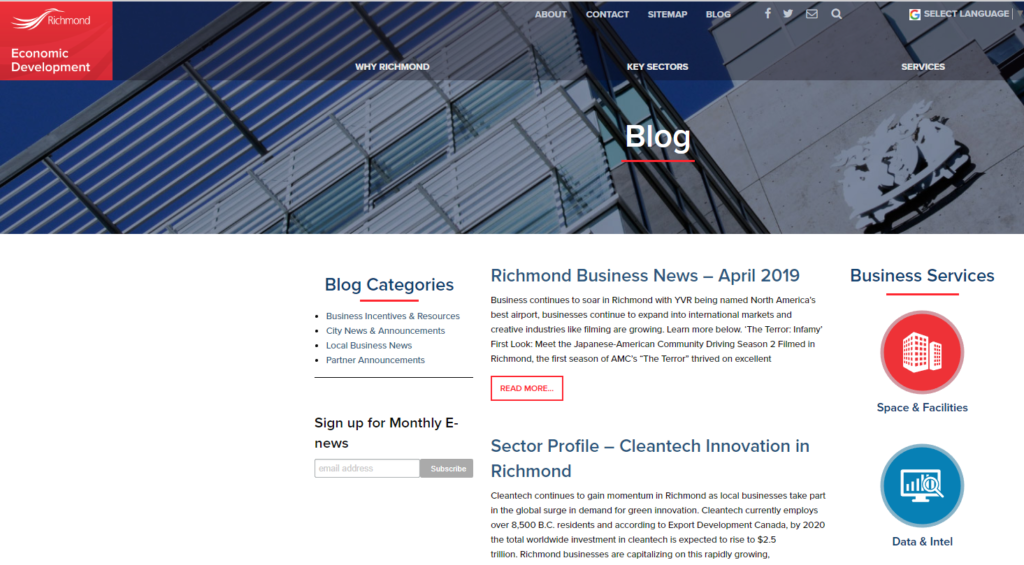The image is a screenshot from a website showcasing a structured layout. The background is divided into two distinct sections: the top third, featuring shades of blue with a photo of the side of a modern skyscraper captured at a diagonal angle, and the bottom two-thirds, characterized by a solid white background.

In the upper left corner, a prominent red square with white text reads "Richmond Economic Development." Centrally positioned in the top section, three category labels—"Why Richmond," "Key Sectors," and "Services"—are displayed in white font. Notably, the word "Blog" appears in a bolder white font in the same central area.

Transitioning to the white background below, the headline "Richmond Business News April 2019" is prominently written in blue. Directly beneath this headline is a paragraph, followed by another headline that states "Sector Profile: Cleantech Innovation in Richmond." This structured format appears to organize and present information clearly to the viewer.